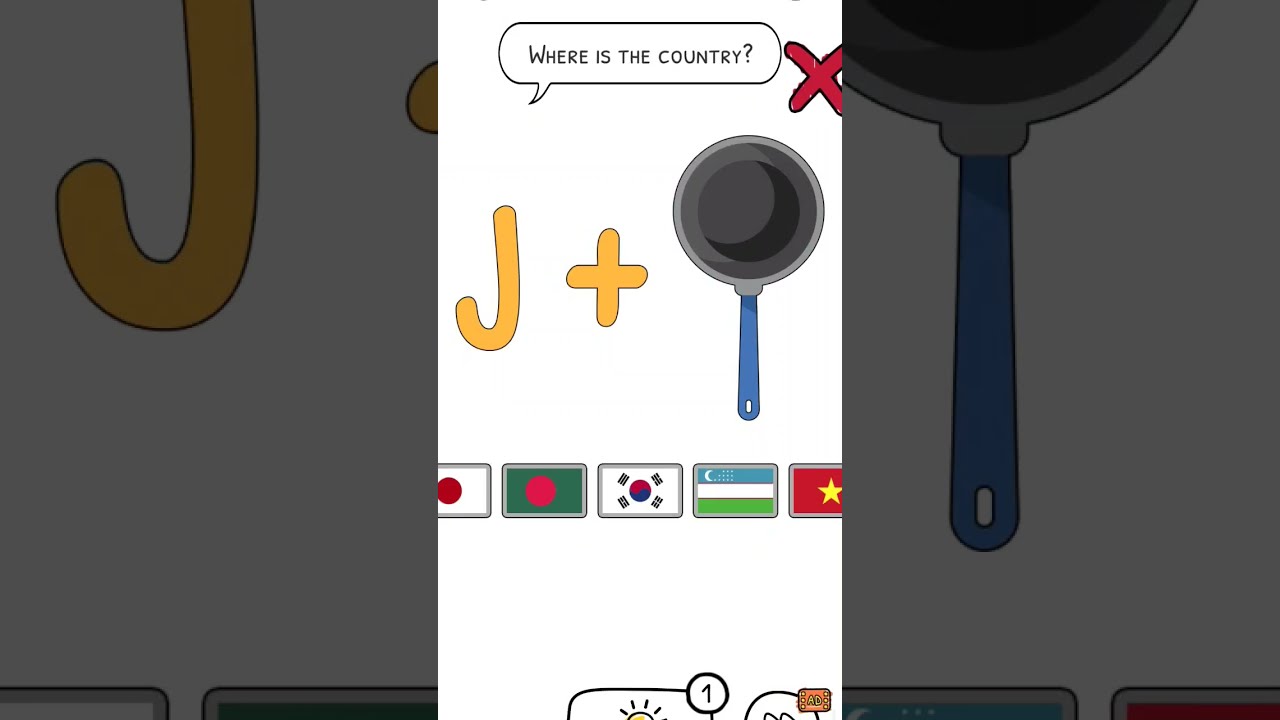The screenshot, taken vertically on a mobile phone, depicts an educational app designed for young children to learn about different cultures and countries. The UI is simple and elementary. The background is white, and the top of the screen features a speech bubble with the question "Where is the country?" accompanied by a red cartoony 'X'. Below this, occupying most of the upper half, is a yellow letter 'J' followed by a plus sign and a cartoon image of a frying pan with a blue handle. Directly beneath this graphic, a series of country flags run horizontally across the screen, featuring flags from Japan, Bangladesh, South Korea, and Vietnam among others. Behind the main content, an enlarged and darkened duplicate of the image with the letter 'J' and the frying pan appears faintly on the left and right sides, giving the illusion of additional layers.